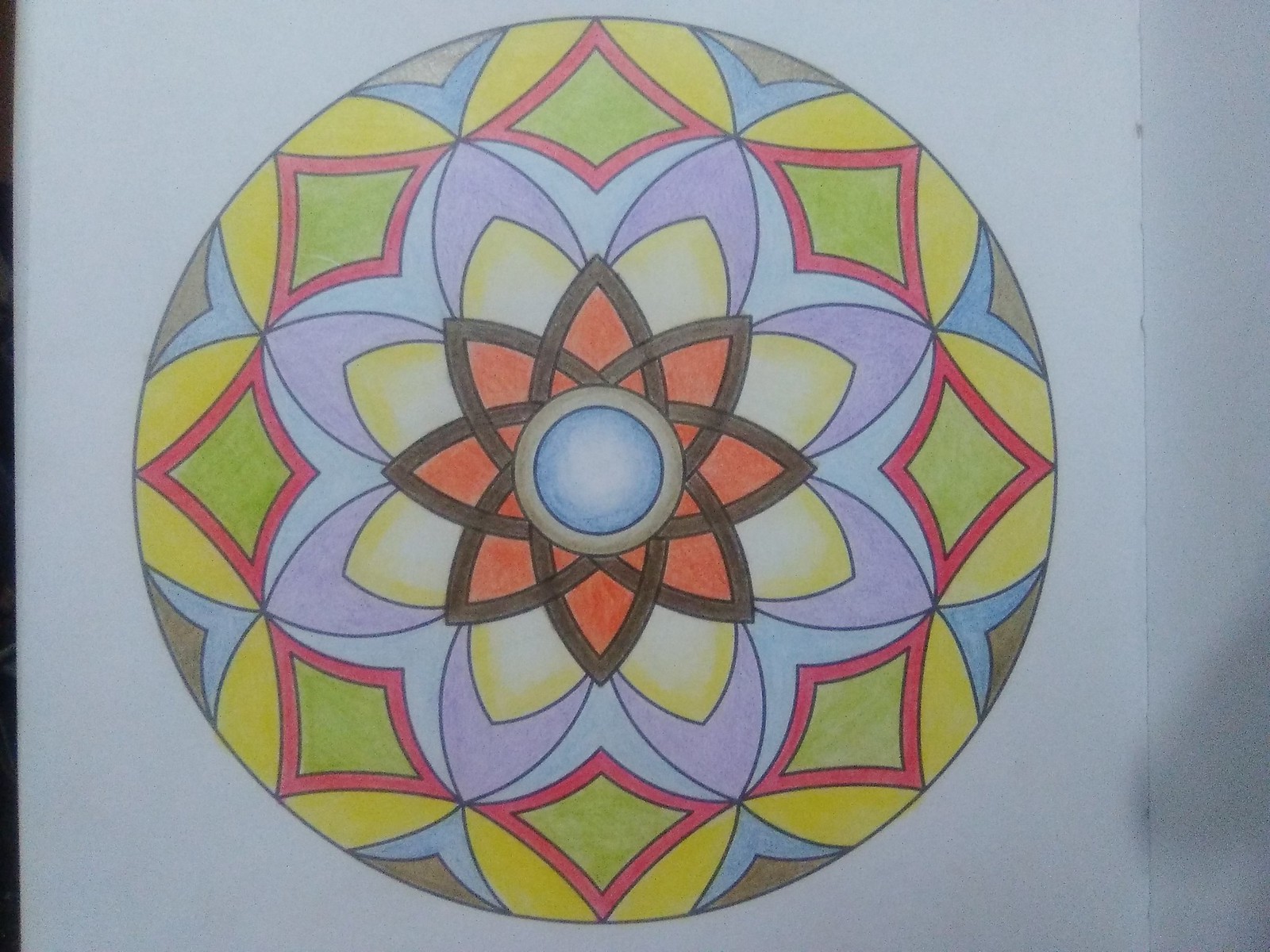This photograph features a detailed, circular drawing with intersecting geometric patterns reminiscent of Middle Eastern tile designs or spirograph art. The artwork is on white paper and appears mounted, possibly on a wall, though there's some ambiguity with visible shadowing on the right side suggesting it might be partially on a table. At its core, a blue circle is surrounded by a gray ring. From this center, eight segments fan out in a flower-like formation, featuring a rich palette of colors, possibly applied with crayons or colored pencils. 

The primary segments adjacent to the center are sharp domed shapes in orange with brown borders, followed by a sequence of yellow, purple, and blue patterns. These colorful segments are complemented by a peripheral arrangement of green diamonds bordered in orange, all touching the outer edges of the design. The intricate layering of colors includes brown, light blue, red, and green hues, among others. The overall image doesn't completely fill the photograph, with its edges cut off on the right, enhancing the impression of a meticulously crafted, vibrant geometric composition.